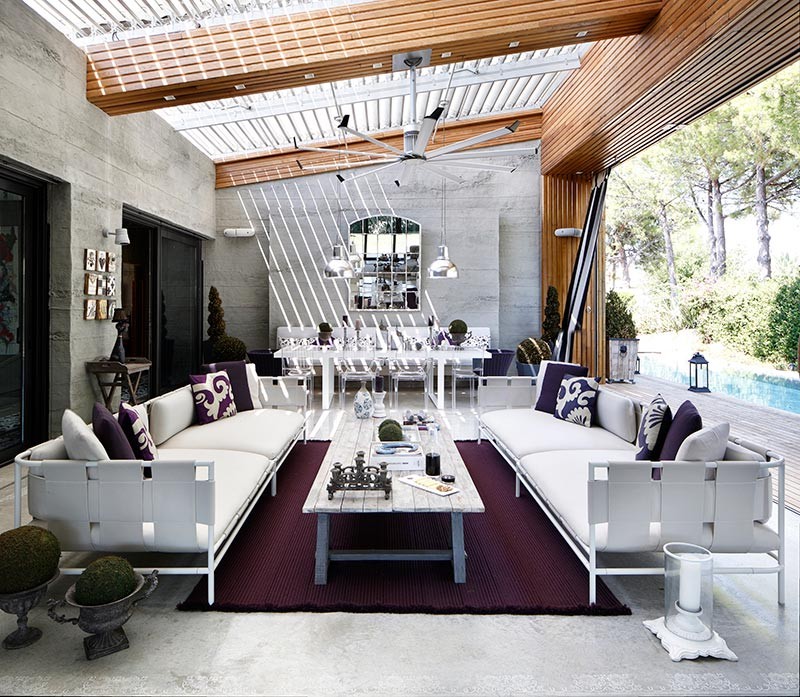This image showcases a beautifully designed sunroom, located on the perimeter of a house, exuding a warm and inviting atmosphere. The sunroom features an impressively large window that dominates the right side, offering a panoramic view of a tranquil outdoor space. Outside the window, a wooden deck extends outwards, leading to what appears to be a long, river-like pool that enhances the serene setting.

Inside the sunroom, the space is elegantly furnished with two sizable couches, positioned on either side of an extended coffee table. A rich burgundy rug partially lies beneath the front of the couches and the table, adding a touch of color and contrast. The decor includes a few distinct items, notably two Roman-style goblets that hold plants, hinting at the likelihood that this is a 3D rendering given their perfectly detailed and slightly exaggerated appearance.

The architectural details of the room stand out, with prominent wooden beams spanning the ceiling and a particularly large beam near the expansive window, contributing to the room's rustic yet refined aesthetic. Sliding doors opposite the large window connect this space to the rest of the house, reinforcing the idea that this is indeed a sunroom—a space meant to blend indoor comfort with the outdoor beauty.